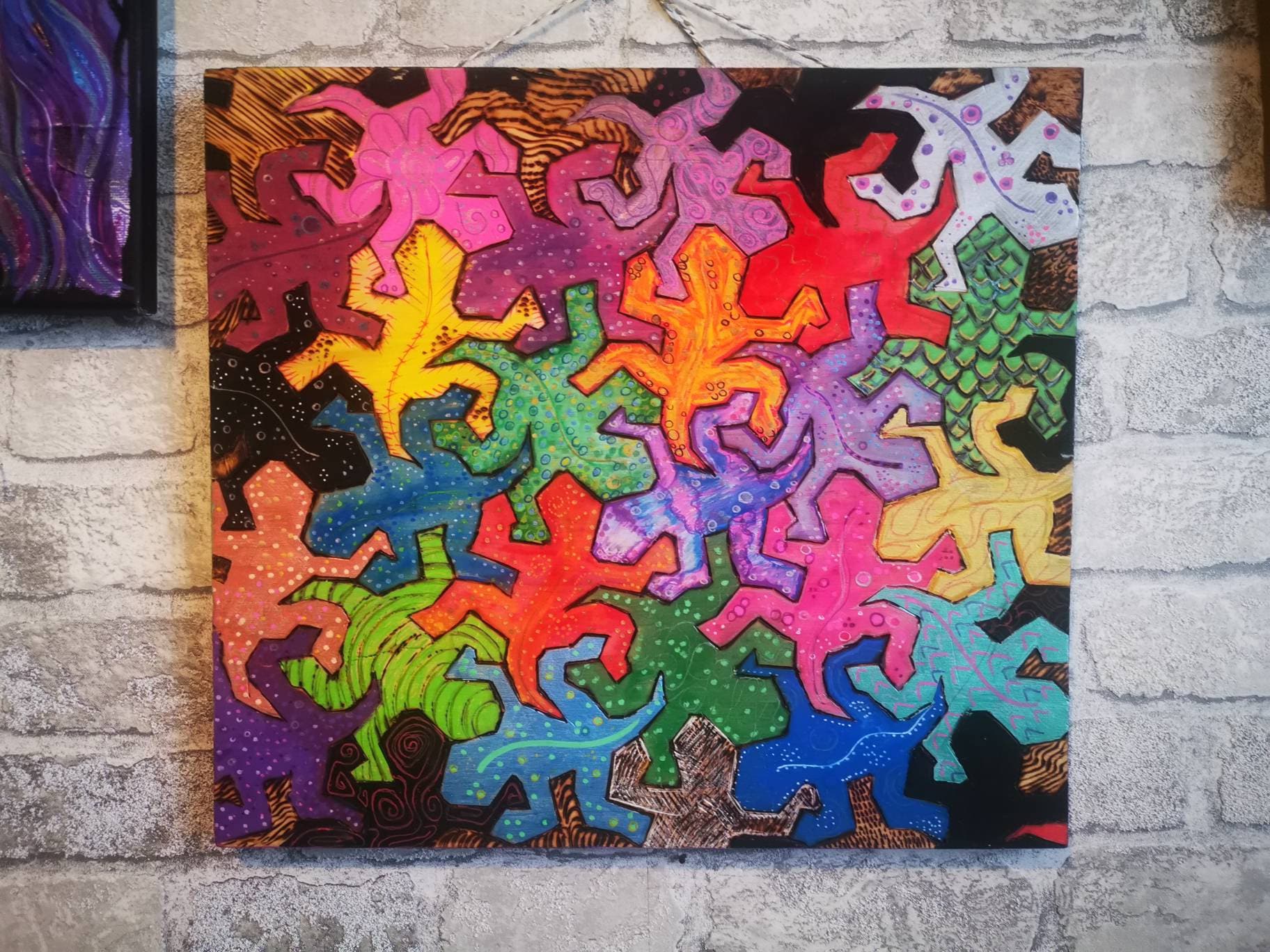This image captures a rectangular, light-colored stone wall, textured to appear like bricks, giving it a slightly gray hue due to the underlying colors bleeding through. The focal point is a large, vibrant canvas painting positioned centrally on the wall. This painting features an interconnected pattern of small, colorful animals reminiscent of lizards or geckos, each adorned with intricate designs such as lines and dots, and arranged like puzzle pieces. The lizards are depicted in a plethora of bright colors—reds, greens, blues, purples, pinks, yellows, and oranges—with variations in shades and decorations creating a lively and dynamic composition. In the top right corner of the wall, there's a small, indistinct brown smudge descending. Meanwhile, the top left corner reveals a partial view of a second framed piece, characterized by a black frame and featuring purple abstract squiggly designs. This secondary artwork adds a subtle hint of additional artistic elements to the overall scene.